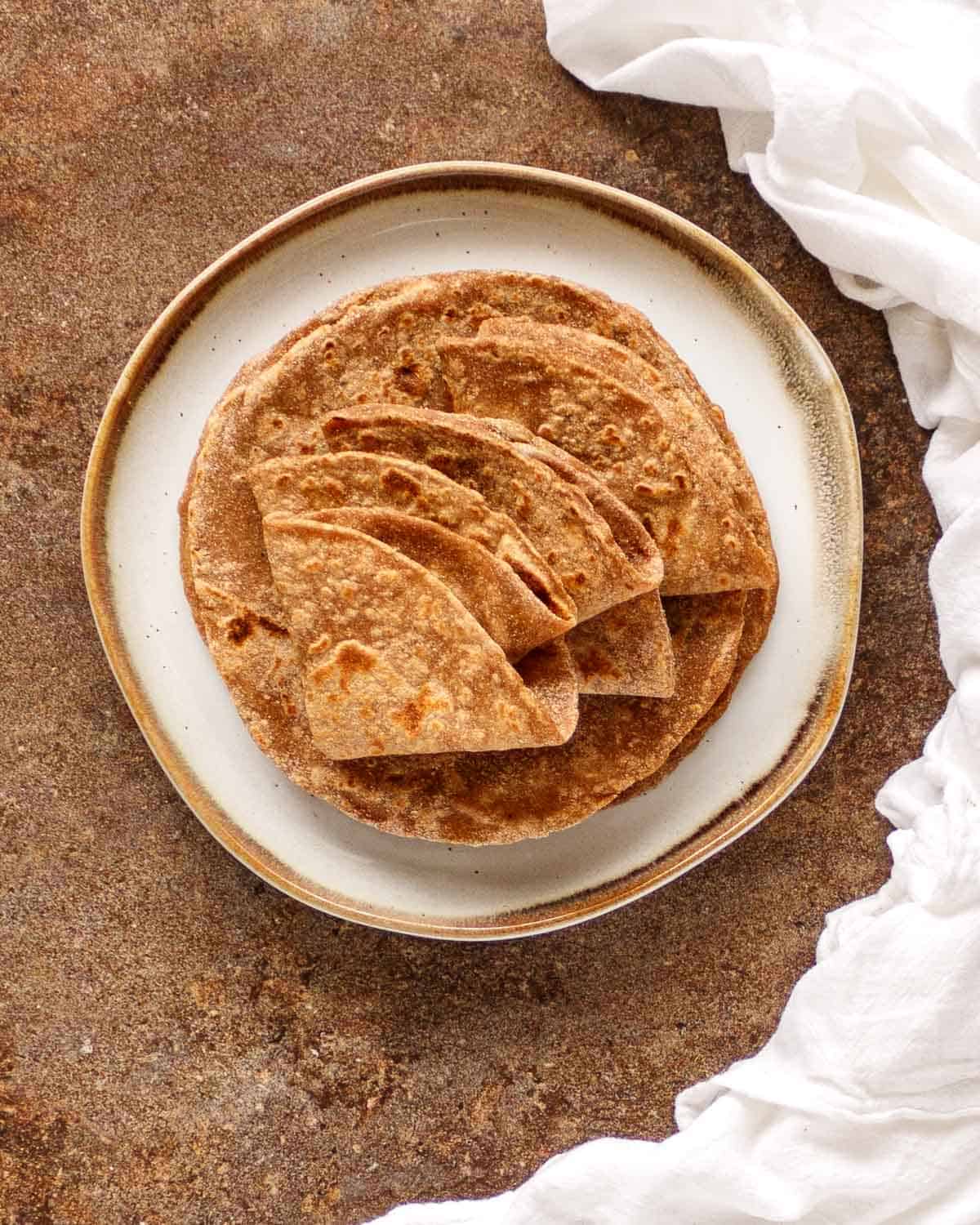The image depicts a charming, rustic ceramic plate with imperfections, giving it a unique, handmade feel. The plate features a white center surrounded by a brown rim and is not a perfect circle. It sits on a surface resembling packed, hard sand or brownstone, with a slightly rough texture. Draped around the edge of the plate is a folded white cloth.

On the plate, there are several pieces of thin, tortilla-like bread. Some pieces are laid flat, while others are folded into quarter shapes, resembling slices of pie. These bread pieces appear toasted, with a light dusting of what could be cinnamon, adding a touch of color and texture. The photograph is taken from a high angle directly above the plate, effectively capturing the quaint and rustic ambiance of the setting.